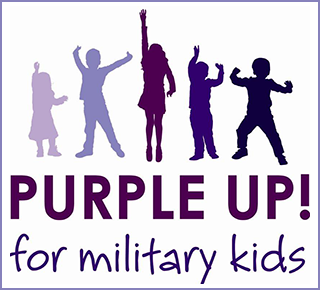The image is a simple yet striking square graphic with a solid white background and a thin purple border. Dominating the upper portion are five silhouettes of children, arranged in a gradient from light purple on the left to nearly black on the right, creating a visually engaging slope. At the center, a girl in a short dress or a long-sleeved shirt and skirt lifts her right arm high, forming a fist. Flanking her are shorter boys, each raising their arms, feet slightly apart - one in light purple and the other in dark purple. To the far left, a very light lavender girl mirrors this uplifted gesture, while to the far right, a boy in the darkest purple does the same, his feet further apart. Below this spirited assembly, bold, capitalized purple letters shout "PURPLE UP!" beneath which, in a playful, lowercase handwriting font, reads "for military kids," underscoring an initiative to support children in military families. Both lines of text span the width of the image, echoing the unity and support signified by the raising arms of the children above.